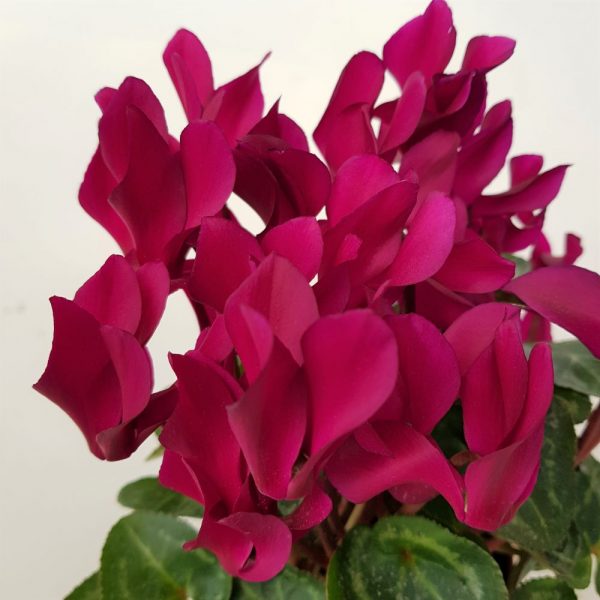This image features a vibrant plant set against a plain white background, emphasizing its colorful and distinct elements. The top two-thirds of the image is dominated by numerous magenta, teardrop-shaped flower buds that cascade downward from the upper portion. These bright flowers capture immediate attention and give a sense of lushness. Beneath the flowers, green leaves with light green striping are visible, varying in size and orientation. Some leaves stand straight up while others are either folded inward, downward, or upward, adding a dynamic texture to the plant. The leaves also exhibit some imperfections, such as one with a tiny hole and another that is brown on the right side of the image. The stems, mostly blurred and barely visible, show a gradient from green to slightly brown as they reach towards the bottom of the plant. The image appears to be cut off at the bottom and the right side, focusing primarily on the vibrant flowers and intricate leaves.